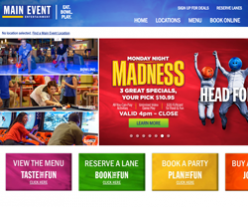The image appears to be a low-resolution, multicolored snapshot of a website dedicated to event promotion and booking. The main background is predominantly white, offering a clean and minimalistic aesthetic. 

At the top, a gradient blue banner spans the width of the page, transitioning from dark blue on the left to a lighter shade in the center, and back to dark blue on the right. On the left side of the banner, the words "MAIN EVENT" are prominently displayed in white capital letters, accompanied by an unreadable yellow text beneath "MAIN." Further to the right within the banner, there are two minuscule, unreadable white texts.

Just below the banner, a row of navigation buttons is visible. The first button is labeled "Home," followed by an unreadable second button. The third button seems to say "Menu," and the fourth one reads "Book Online" in white text.

Beneath this navigation, a white bar serves as the main content area, featuring very small black text that is too tiny to decipher. This is followed by three horizontally stacked landscape images, each depicting different scenes: 

- The top image, predominantly blue, appears to feature two individuals.
- The middle image also seems to include people.
- The bottom image shows what looks like a man and a woman engaged in some activity.

To the right of these images, there is a large red block with the word "MADNESS" in yellow text, followed by illegible smaller text about specials and a green button beneath it.

Adjacent to this red block, an image shows a man and a woman mid-jump, possibly wearing bodysuits or Formula 1 racing suits, characterized by red and blue heads. Above this image, the text "HEAD FOR" is partially visible.

At the very bottom of the page, four rectangular buttons offer various calls to action:
1. "View the Menu, Taste the Fun" on a purple background.
2. "Reserve a Lane, Book the Fun" on a green background.
3. "Book a Party, Play for Fun" on a yellow background.
4. "Buy [Unreadable]" on an orange background. 

Overall, the website presents a vibrant and dynamic design aimed at promoting events and activities, despite the fuzziness of the image.